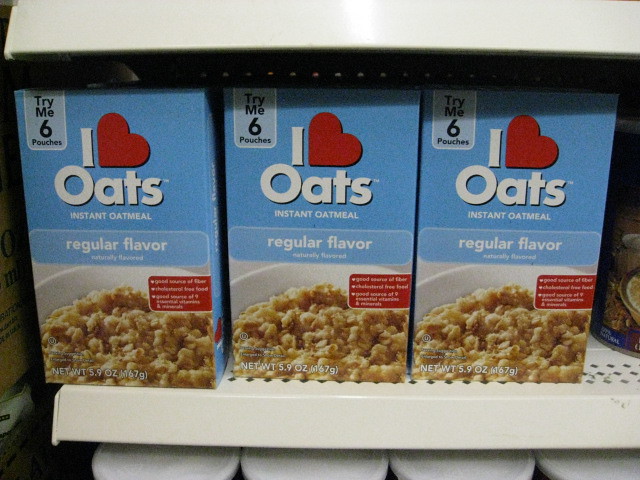This image depicts a grocery store shelf stocked with three identical light blue boxes of "I Love Oats Instant Oatmeal." The boxes prominently feature a red heart symbol representing the word "Love" in the product name. Each box includes the phrase "Try Me 6 Pouches" in black lettering near the top left corner. Below the product name, "Instant Oatmeal" is printed in smaller white lettering above a blue rectangle with the words "Regular Flavor, Naturally Flavored." A partial image of a bowl of beige oatmeal is visible at the bottom right, right below the flavor description. Near this bowl, there's a red box with white letters highlighting nutritional benefits, including "Good Source of Fiber" and "Cholesterol Free," though some text is illegible. The boxes state the net weight as 5.9 ounces (67 grams) at the bottom left corner. The middle box is slightly pulled out compared to the others. They sit on a white shelf with a series of diamond-shaped holes forming a pattern across the shelf's front. Below this shelf, four partially visible white circular lids can be seen. The image captures natural fluorescent lighting, amplifying the visibility of the products and the store shelf details.